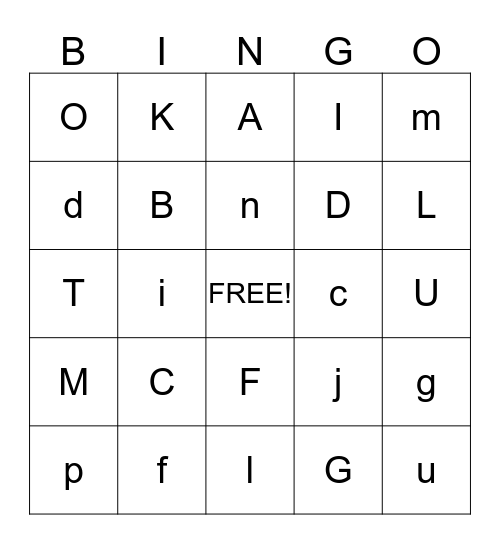The image features a bingo card with a white background and the word "BINGO" in black text across the top. The card is structured in a 5x5 grid, with each column labeled by one of the letters of "BINGO". Some letters in the grid are capitalized while others are in lowercase. The B column contains letters O, D, T, M, and P (with D and P in lowercase). The I column holds letters K, B, I, C, and F (I and F in lowercase). Under the N column, which includes the free space, are letters A, N (lowercase), and F, I. The G column has I, D, C, J, and G (C and J in lowercase). Finally, the O column features M, L, U, G, and U (G and last U in lowercase). The center square prominently displays the word "FREE!" in capital letters with an exclamation point.